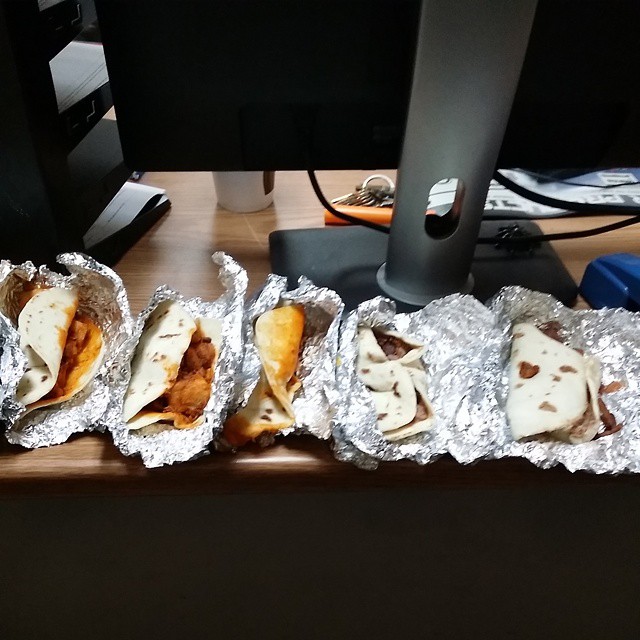This is an indoor color photograph showcasing a wood-toned brown desk featuring five flour tortillas neatly wrapped in tinfoil, all opened to reveal their contents. The tacos stretch across the middle of the image, from left to right, with each individual foil packet visibly crinkled. The tortillas are white with brown spots and various fillings peek out, including what appears to be meat in some and a pale brown bean mixture in others. The leftmost taco has an orange filling spilling out slightly. Situated behind the tacos is the backside of a black and silver rectangular computer monitor, its stand extending down beneath the tacos. Also resting on the desk are a set of car keys and a glimpse of a coffee cup.